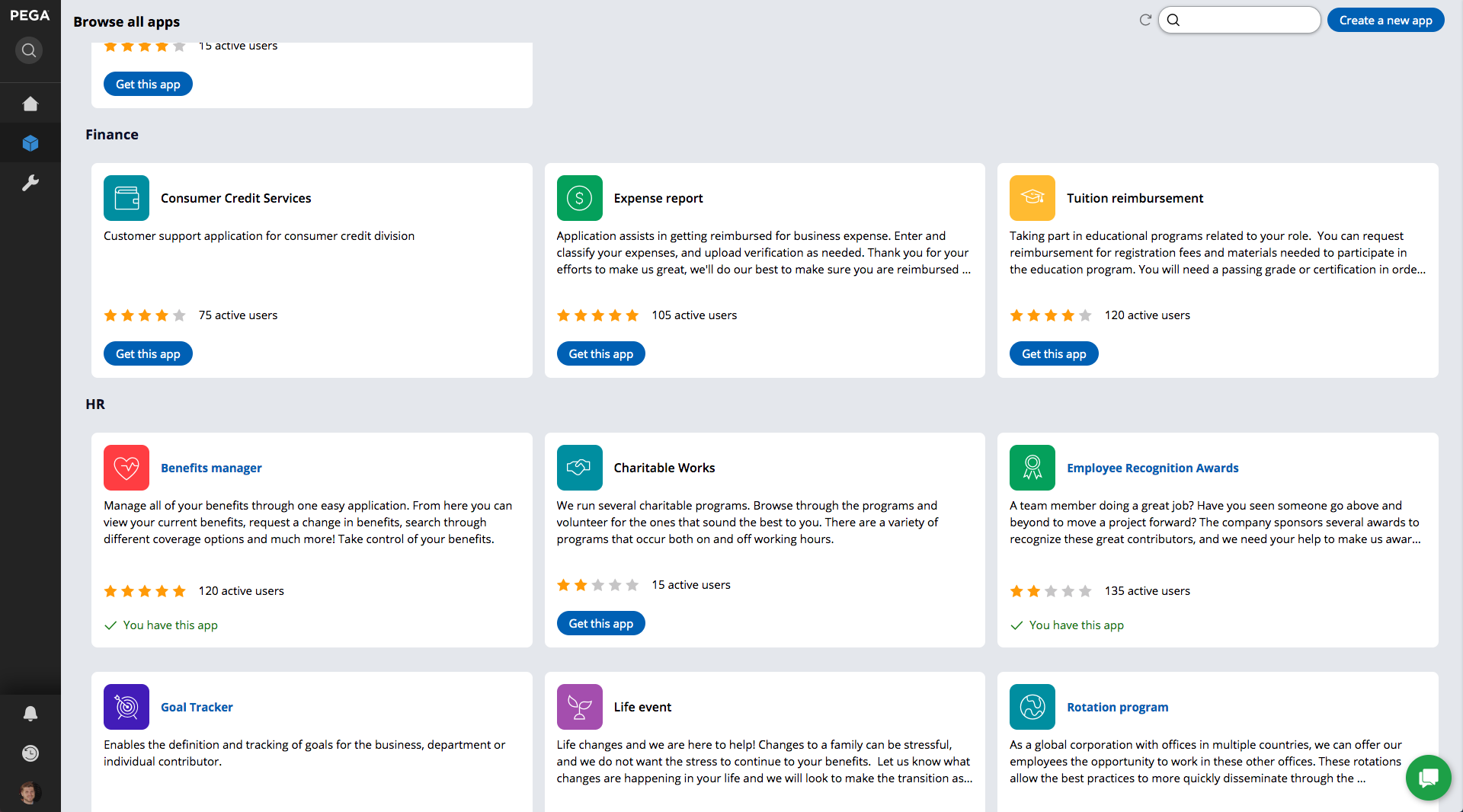The screenshot showcases the interface of a business application directory, potentially hosted by a company named PEGA. On the far left, there is a narrow sidebar featuring the company's logo "PEGA" at the top, followed by a small search bar for navigating the site. Below the search bar, icons such as a home page link, a wrench symbolizing tools or settings, and various alert notifications are visible.

The main section of the page is dedicated to browsing available applications, sorted into different categories. At the top left, the "Finance" category is highlighted, listing apps like "Consumer Credit Services" and "Customer Support Application." Each app description includes details such as user ratings and specific features—one, for example, has "75 active users" and offers assets for managing business expenses and tuition reimbursement for educational programs.

Further down, the screenshot displays other categories like "HR." Under HR, it lists benefits like "Goal Tracker," the "Life Event Rotation Program," and applications for employee perks such as "Benefits Manager," "Charitable Works," and "Employee Recognition Awards." The status of each app is indicated, showing whether the user already has the app or not, with green checkmarks denoting active applications.

Overall, the screenshot depicts a structured and interactive interface designed to help users explore and manage various business applications provided or aggregated by PEGA.